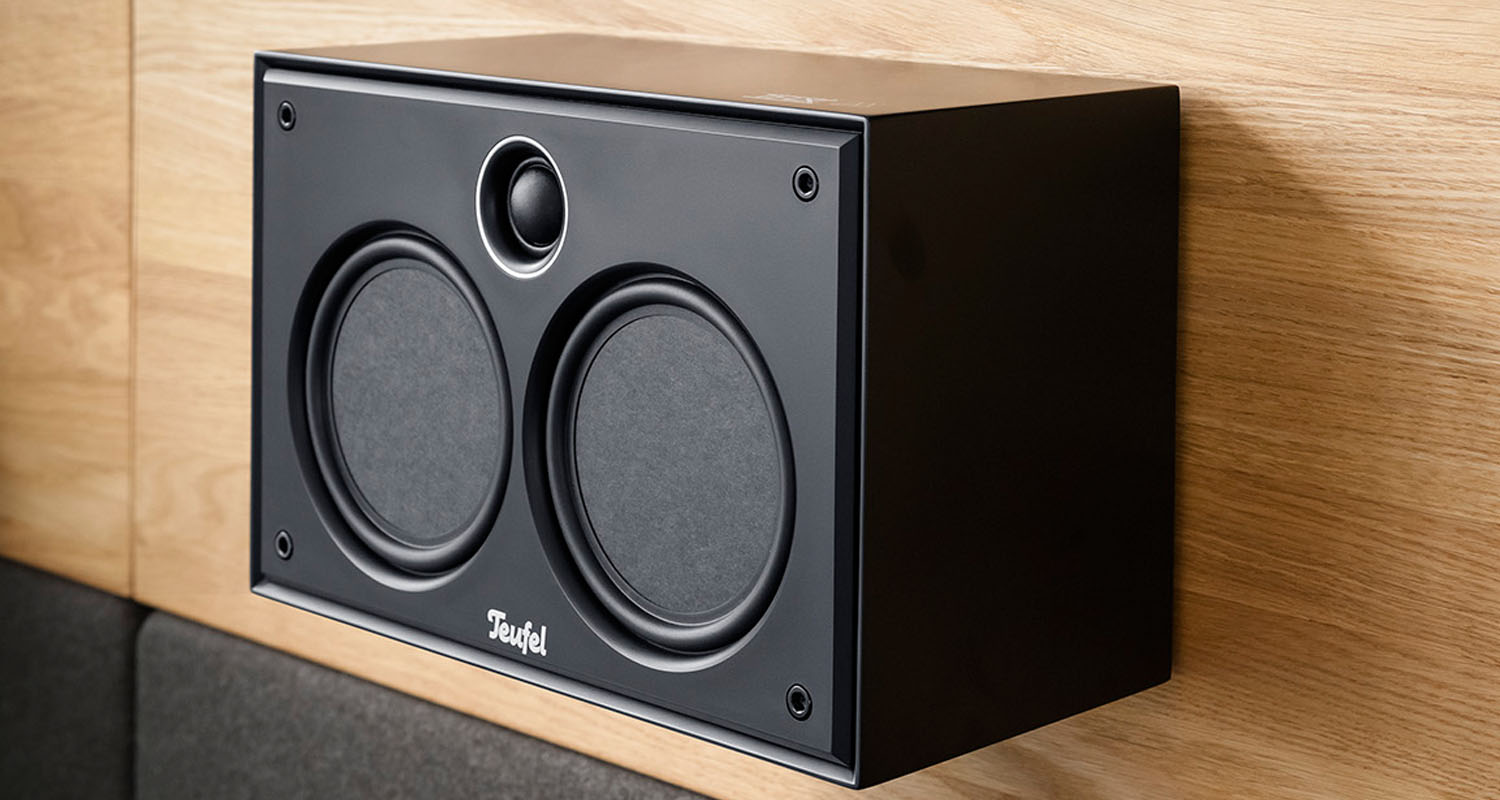This highly detailed photorealistic image showcases a black speaker mounted on a light wood grain panel wall. The speaker features the brand name "TEUFEL" in white font centrally located at the bottom front. The speaker design includes two large, black subwoofers with flat cones, flanking a centrally positioned dome-shaped mid-range speaker or tweeter. Each corner of the speaker has holes designed for an optional cover, though the cover is not depicted. The area below the wooden panel appears to be a wall covered in sound-absorbing cloth material, hinting at an acoustically optimized environment.